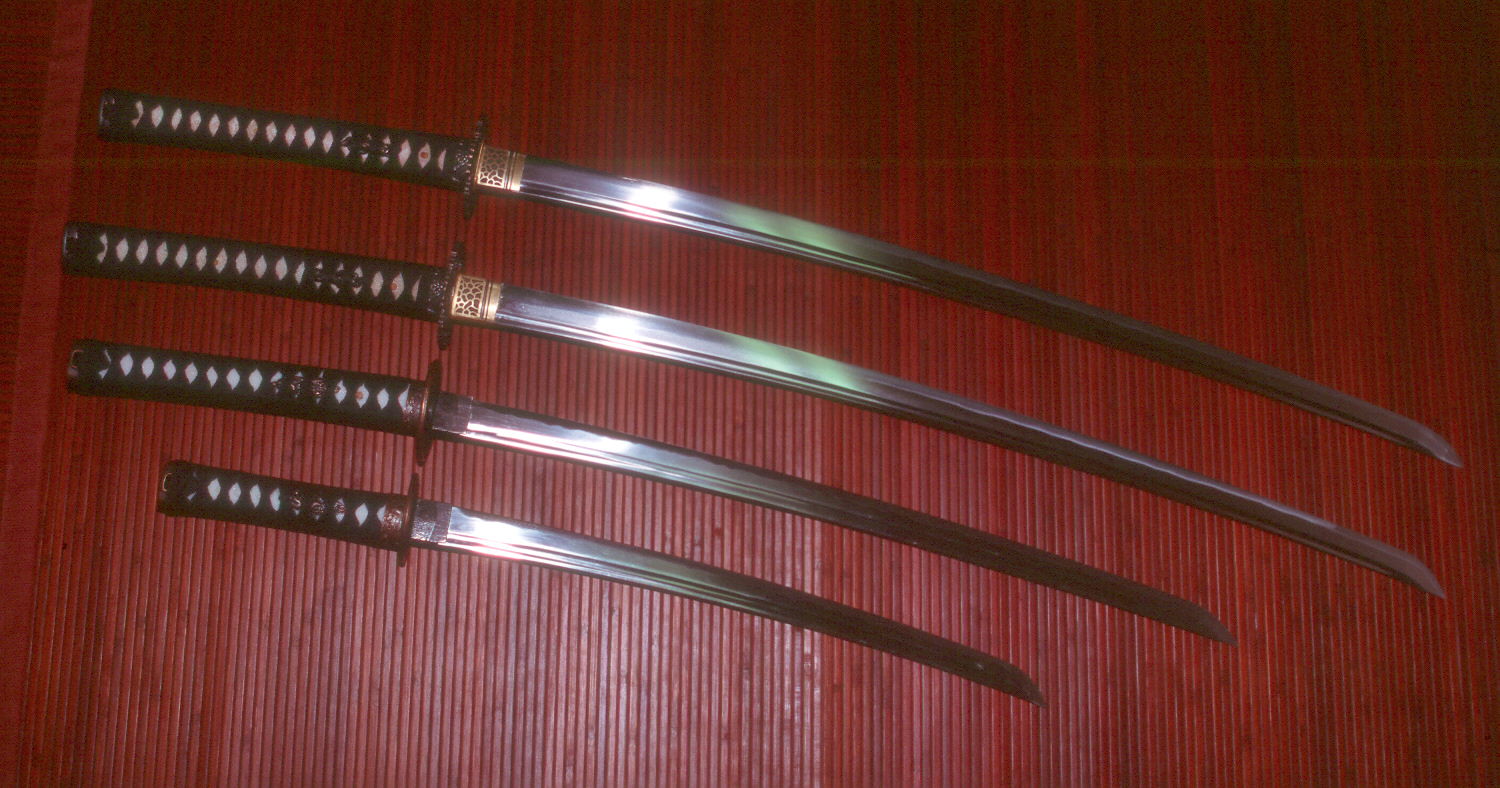This is a color photograph taken indoors, featuring four swords laid out on a reddish, cherry wood-like paneling. The background comprises thin vertical strips of reeded wood, adding texture to the image. The swords are arranged in a neat row, all facing the same direction with the blades visible from handle to tip.

The first two swords at the top are identical and very long, each equipped with a black handle and a silver blade. At the point where the blade meets the handle, there's a small golden emblem that adds a touch of detail. The third sword is slightly shorter but shares the same design elements as the top two, including the black handle and the silver blade. The fourth and shortest sword also mimics the design of the others, with a black handle highlighted by a red emblem and a shining silver blade. Light reflects off the blades, adding a bright, shiny appearance to parts of the swords. Each handle features distinct white shapes, providing a subtle but noticeable contrast to the black.

Overall, the photograph captures the uniformity and detailed craftsmanship of the four swords against the rich, warm backdrop, emphasizing their similar yet varying lengths and intricate design.